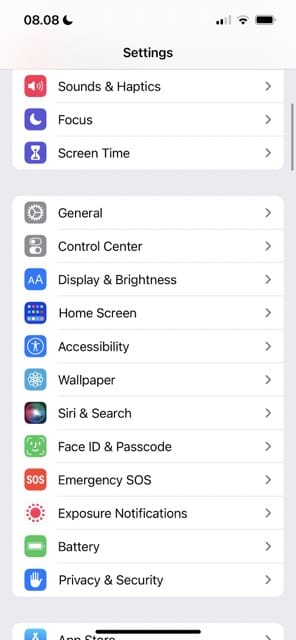This image depicts a screenshot of the "Settings" menu on a mobile device, likely from an Android or iPhone, in a portrait orientation. 

At the very top, there is a faint gray rectangular status bar. On the upper left of this bar, the time is displayed as "08:08" next to a partial black and white clock icon. On the upper right, there are two out of four signal bars, a Wi-Fi icon, and a fully charged battery icon, all in black and white.

Below the status bar, centered, the word "Settings" is written in bold black letters. Following this header, there are several segmented menu options, each accompanied by an icon to the left and a description to the right, along with a sideways-facing "V" indicating these options can be expanded:

1. **Sound:** Represented by a red square with a white speaker volume icon.
2. **Focus:** Displayed with a purple box containing a white moon icon.
3. **Screen Time:** Shown with a purple square with a white hourglass icon.
4. **General:** Depicted by a gray square with a white circle containing a peace sign-like icon. 
5. **Control Center:** Represented by a gray square with a toggle switch icon.
6. **Display & Brightness:** Indicated by a blue square featuring two capital A's, the right one larger, in white.
7. **Home Screen:** Marked with a blue square containing multicolored dots.
8. **Accessibility:** Shown with a lighter blue square and a white person icon.
9. **Wallpaper:** Depicted by a faint blue square with a white rose icon.
10. **Siri & Search:** Represented by a black square with a multicolored circle.
11. **Face ID & Passcode:** Marked with a grass green square featuring a white smiling face icon.
12. **Emergency SOS:** Illustrated by a red box with "SOS" in white capital letters.
13. **Exposure Notifications:** Shown with a red circle surrounded by red dots resembling a sun icon.
14. **Battery:** Represented by a grass green square with a faint blue blurry bar.
15. **Privacy & Security:** Indicated by a blue square with a white hand icon, palms out.

At the bottom of the screenshot, there is a long thin black bar centered in the gray area. Below this, the top of the next white area is visible, showing part of another blue box on the lower left with a partially visible white symbol and text that gets cut off.